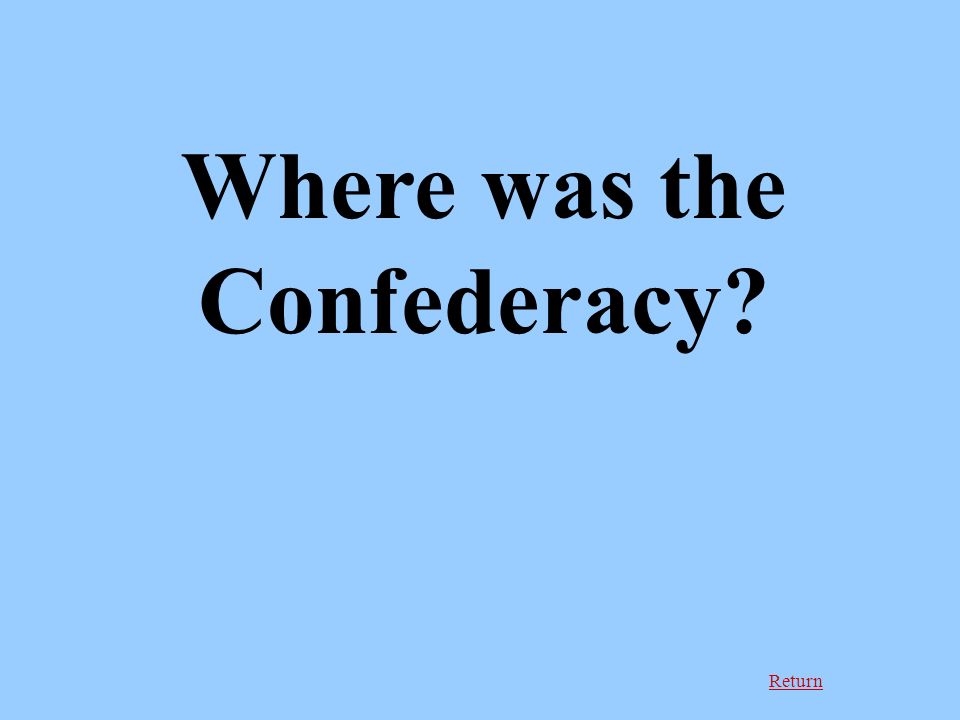The image is a square, light blue slide that seems to be part of a presentation or slideshow. The central focus is on the black text, split into two lines: "Where was the" on the first line and "Confederacy?" on the second line. In the bottom right-hand corner, there's an underlined "return" button in red, suggesting it serves as a hyperlink to navigate back to a previous slide. The slide is simple and uncluttered, designed purely to pose the question, with no additional elements or watermarks.